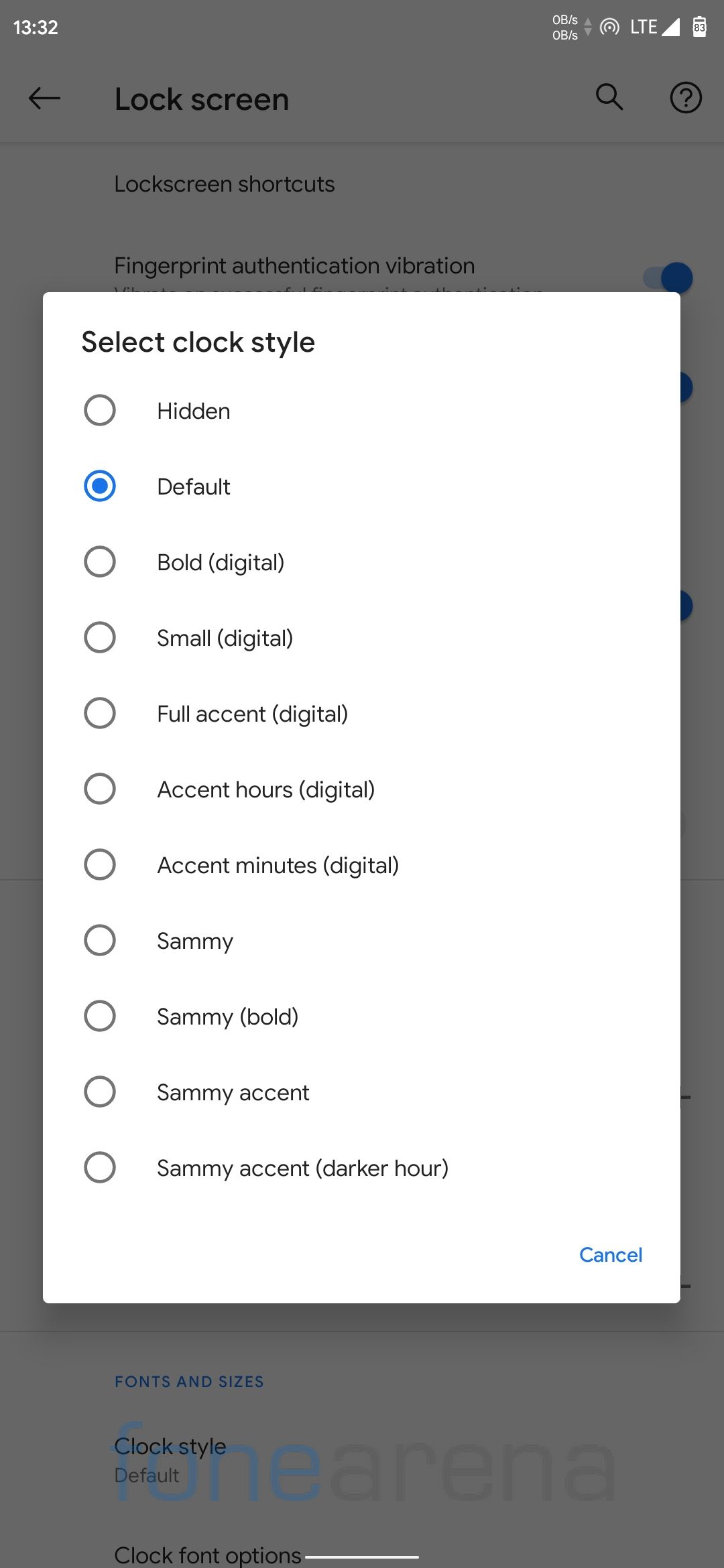The image shows a smartphone screen displaying the device's settings menu, with an overlaying pop-up window. The background is grayed out, indicating that the settings page is inactive while the pop-up is being interacted with. The screen time is 13:32, and the status bar shows LTE signal strength with full bars, an 83% charged battery, and data sharing indicators. 

The grayed-out settings screen underneath displays headings like "Lock Screen," "Lock Screen Shortcuts," "Fingerprint Authentication," and "Vibration," although these options are partially obscured by the pop-up window. 

The pop-up window, predominantly white with black font, presents a list of clock style options for the lock screen. Each option is accompanied by a circular radio button, with the currently selected one highlighted in blue. The list includes "Hidden," "Default" (which is currently selected), "Old Digital," "Small Digital," "Full Accent Digital," "Accent Hours," "Accent Minutes," "Sammy," "Sammy Bold," "Sammy Accent," and "Sammy Accent Darker Hour." 

In the bottom right corner of the pop-up, there is a blue "Cancel" button. The bottom-left corner of the screen includes a faint watermark reading "Phone Arena," with "Phone" in blue text and "Arena" in gray text.